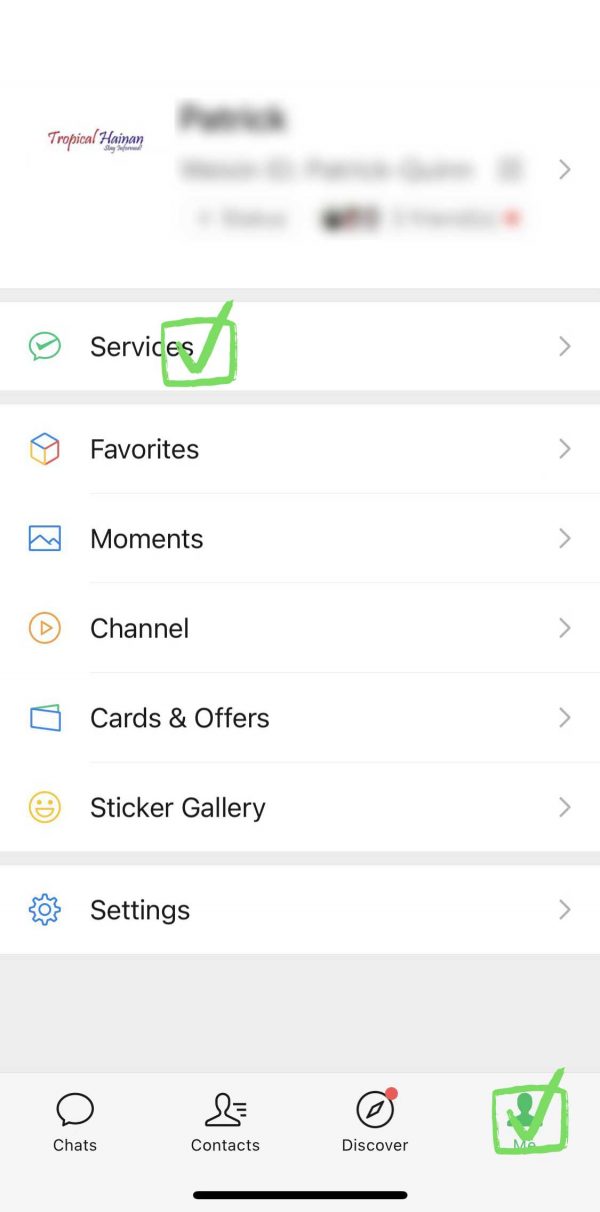This image, magnified to 200%, reveals a variety of intricate details, though some elements remain indistinct. In the upper left corner, the word "tropical" is written in red cursive script, and "hajman" appears in black. Adjacent to this, three lines of text seem to be deliberately obscured, either blacked out or blurred. Below these lines, the word "services" is visible, accompanied by a green checkmark. This checkmark looks as though it has been manually drawn within a green box.

Moving down the image, the term "favorites" appears next to a box, followed by an icon labeled "gallery" that says "moments." Continuing downward, "channel" appears alongside a button symbol, then an envelope icon with the text "cards and offers." A smiley face icon labeled "sticker gallery" follows, and a small tool icon indicates "settings." The options "chats," "contacts," and "discover" are listed, with another manually drawn green checkmark on the right side, mirroring the one seen near "services." The intricate details suggest a thoughtfully designed, albeit obscured, interface or document.